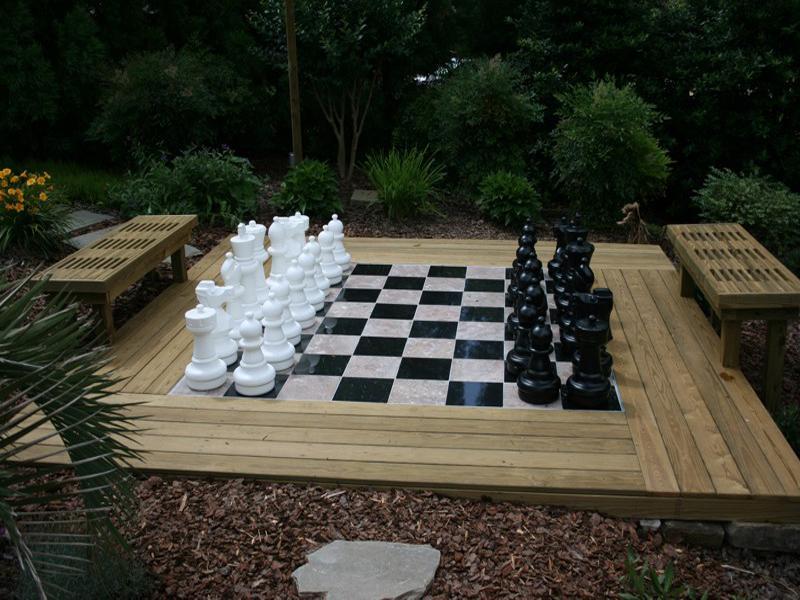This is an outdoor setting featuring a life-size chessboard, appearing to be situated in a well-manicured park or possibly a spacious, beautifully maintained backyard. The chessboard itself is set atop a wooden platform and exhibits a traditional black-and-white tiled pattern. On either side of the chessboard, there are two open-slatted wooden benches that match the wooden flooring surrounding the setup, allowing ample space for players to walk around and move the oversized chess pieces. The white pieces are positioned on the left, while the black pieces occupy the right, with each piece about as tall as or slightly larger than the benches. The area is lush with greenery, including meticulously trimmed bushes, shrubs, neatly planted evergreen trees, and a patch of vibrant yellow wildflowers to the left. The surroundings also feature a stepping stone set in mulch, enhancing the picturesque, park-like atmosphere, although no people are present in the scene.